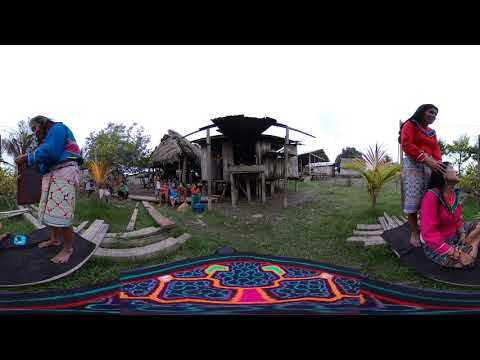The image depicts an outdoor scene centered around a rustic wooden hut with a roof made of hay, flanked by two wooden posts supporting an arched beam. The hut is situated in a grassy area, with patches of rock and dirt visible on the ground. In the foreground, at the bottom of the image, there is a vibrant, colorful mat or rock featuring a square pattern with blue lines and an orange outline. 

To the left of the hut, a barefoot woman wearing a long-sleeved blue top and a white and red patterned skirt stands on a black surface, looking leftwards. On the right side, another woman in a red long-sleeved shirt and white, colorful pants stands, massaging the head of a seated woman in a dark pink shirt and patterned skirt. The seated woman has long black hair. In the background, there are four indistinct figures sitting on a bench in front of the hut. The picture has a horizontal rectangular alignment with thick black borders at the top and bottom, and it seems to have been taken in the middle of the day, likely in an outdoor setting. The scene is brimming with colors such as green, blue, orange, pink, purple, white, red, and gray, enhancing the vibrant and lively atmosphere of the image.